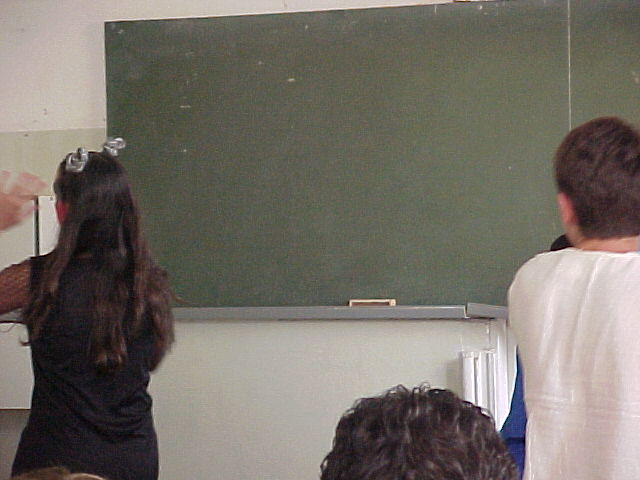This rectangular, landscape-oriented photograph captures a classroom scene from the perspective behind several students. On the left side of the image, a female student with long brown hair is visible, wearing a black shirt and adorned with two earrings. Her left arm extends out of the frame and then reappears within it. Dominating the background is a green chalkboard, nearly spanning the entire width of the image. On the chalkboard's tray rests an eraser, while faint chalk marks are discernible in the upper left corner. To the right, a male student with brown hair wears a white shirt, and the top of another student's dark-haired head is partially visible. The wall behind the chalkboard is painted white, providing a stark contrast to the scene.